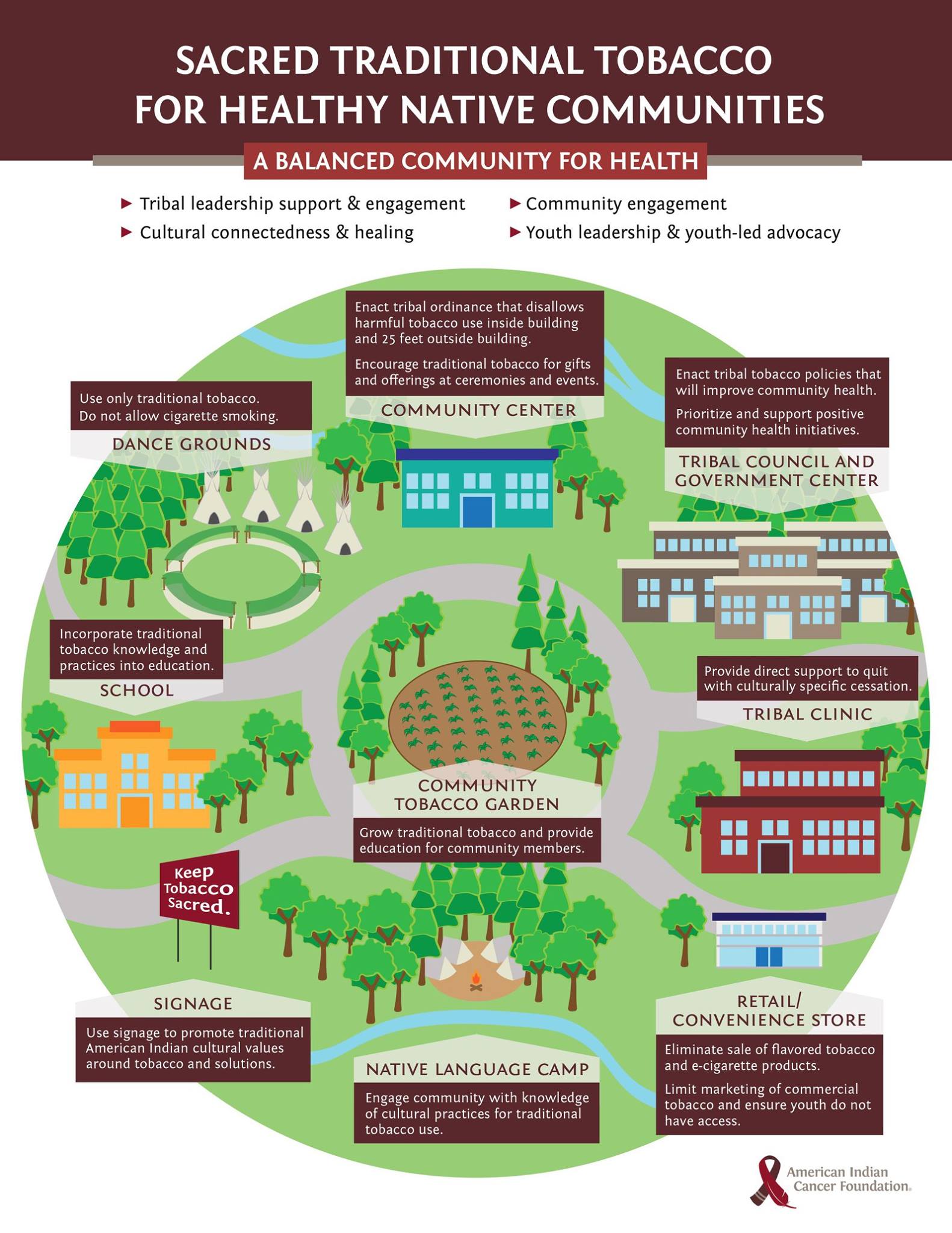The pamphlet features a detailed and vibrant design centered around the theme of "Sacred Traditional Tobacco for Healthy Native Communities." At the top, a burgundy banner with white text enunciates the message, "A Balanced Community for Health." Beneath this heading, several bullet points expound on the tenets of a healthy community.

Dominating the center of the pamphlet is a green circle, illustrating various community areas essential to the well-being of native communities. These areas include:
- Dance Grounds
- Community Center
- Tribal Council and Government Center
- Tribal Clinic
- Retail Convenience Store
- Native Language Camp
- Community Tobacco Garden
- Signage
- School

Each section is accompanied by corresponding images that depict these communal spaces, further emphasizing their importance. The images and text collaboratively highlight the role of traditional tobacco in fostering a healthy, balanced community.

In the bottom right-hand corner, adorned with a ribbon symbol, the pamphlet credits the American Indian Cancer Foundation for their involvement and support in promoting these health initiatives.